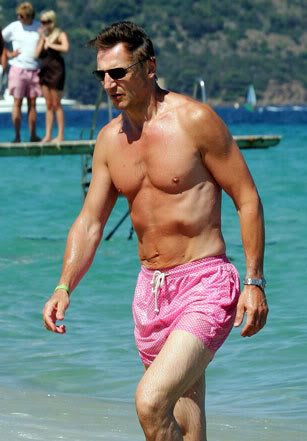The photograph, likely taken candidly outdoors, captures a shirtless Liam Neeson emerging from the water at a sea or lake. He is clad in pink swim trunks with white polka dots and a drawstring, along with a silver watch on his left wrist and a light green band on his right. Neeson’s dark brown hair, brushed to the side, appears dry, suggesting he did not fully submerge himself. He sports black sunglasses and looks downward, showing defined, though modest, muscle tone, with a noticeable tan on his upper body contrasting his lighter legs. In the background, there is a wooden pier to the left with a few people: a blonde woman in sunglasses, a black swimsuit, and a black cover-up, standing next to a blonde man in pink shorts and a white t-shirt, both individuals looking elsewhere. Further behind, a boat and a sailboat are visible on the bright blue water, with a densely vegetated hillside and shoreline in the distance.